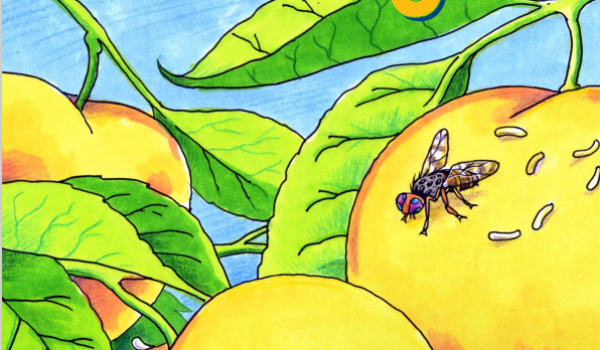This image is a colorful cartoon drawing set against a blue background resembling the sky with faint white clouds and thin, diagonal blue lines adding a window-like effect. The image features green, long oval-shaped leaves adorned with thin black veins, hanging from branches. Among the foliage, there are several fruits in shades of orange and yellow with hints of dark, dull red around the edges, resembling apples. On the rightmost fruit, a detailed fly is perched, characterized by blue eyes, an orange face, a gray back, white-cream wings, and orange legs. Additionally, tiny white and yellowish worms are visible on the same fruit, adding to the intricate details of the scene. With no text present, the vibrant artwork, possibly painted by hand or created digitally, fills the entirety of the vertically arranged rectangular frame.